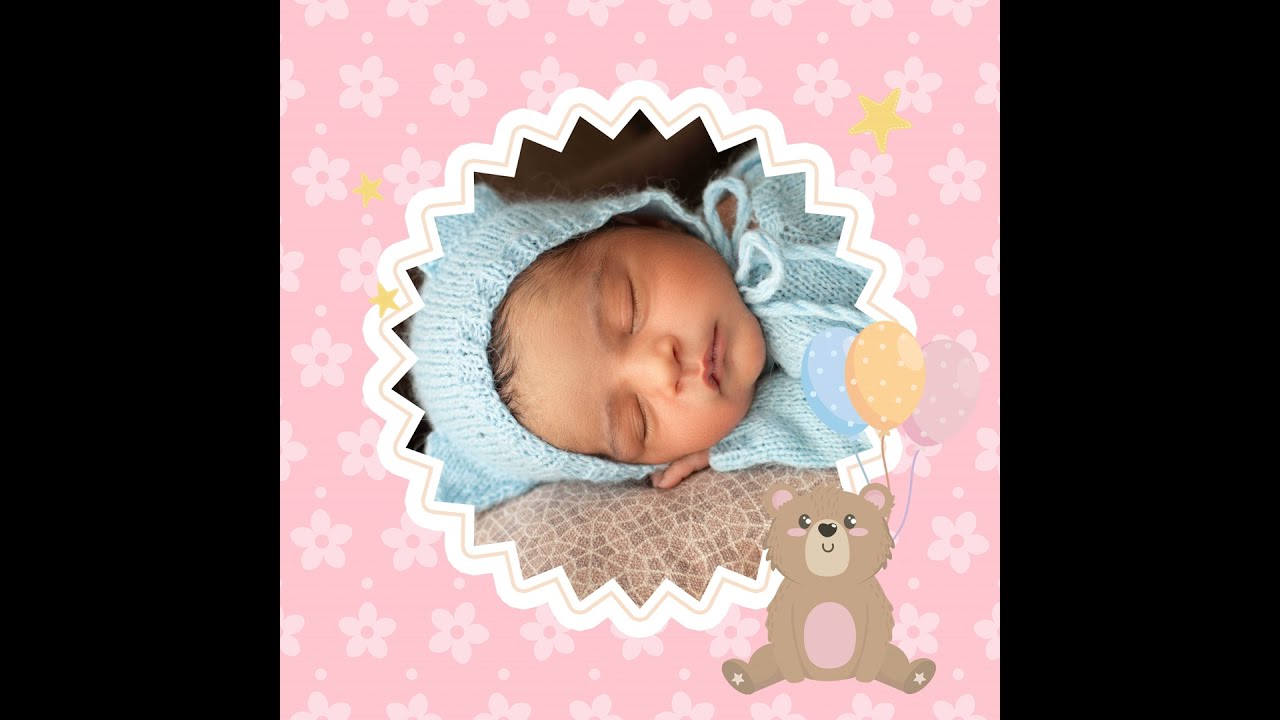This horizontal rectangular image appears to be a birth announcement or greeting card and features a central pink square with a floral background. Flanking the pink square are two thick vertical black borders, each occupying about 20% of the total width of the image. The pink square is adorned with small roses and contains a zigzag-edged white circle with delicate ruffles, serving as a frame for the photograph within.

In the center of this ruffled circle, a sleeping newborn baby is pictured, dressed in a matching light blue hat and onesie. The baby's head is turned slightly to the right, exposing a peek of hair beneath the cap. The infant rests comfortably on a soft, grayish-brown blanket that appears as a gentle cradle.

In the bottom right corner of the central circle, a cute brown teddy bear with a pink belly is illustrated, adding a charming touch; the bear is holding three colorful balloons—blue, yellow, and pink.